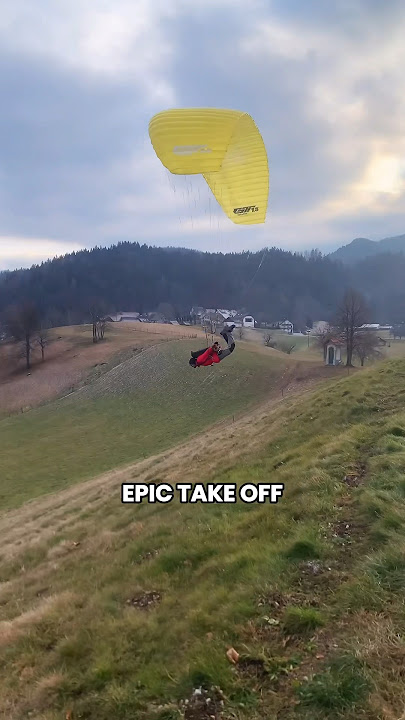This vertical color photograph vividly captures a thrilling outdoor scene of a person paragliding over a green, sloping hillside. The sky above is painted with a mix of blue and white, scattered with gray and white clouds. In the background, dense forests and mountains rise majestically, offering a picturesque backdrop. In the foreground, lighter green rolling hills dotted with patches of dried, yellowish grasses gently lead the eye to the central figure. Wearing a red jacket, the individual is suspended in mid-air, horizontal, under a large yellow parachute. Below the parachute, bold white capital letters with a black outline spell out "Epic Takeoff," suggesting an adventurous leap from the hilltop into the scenic expanse below.